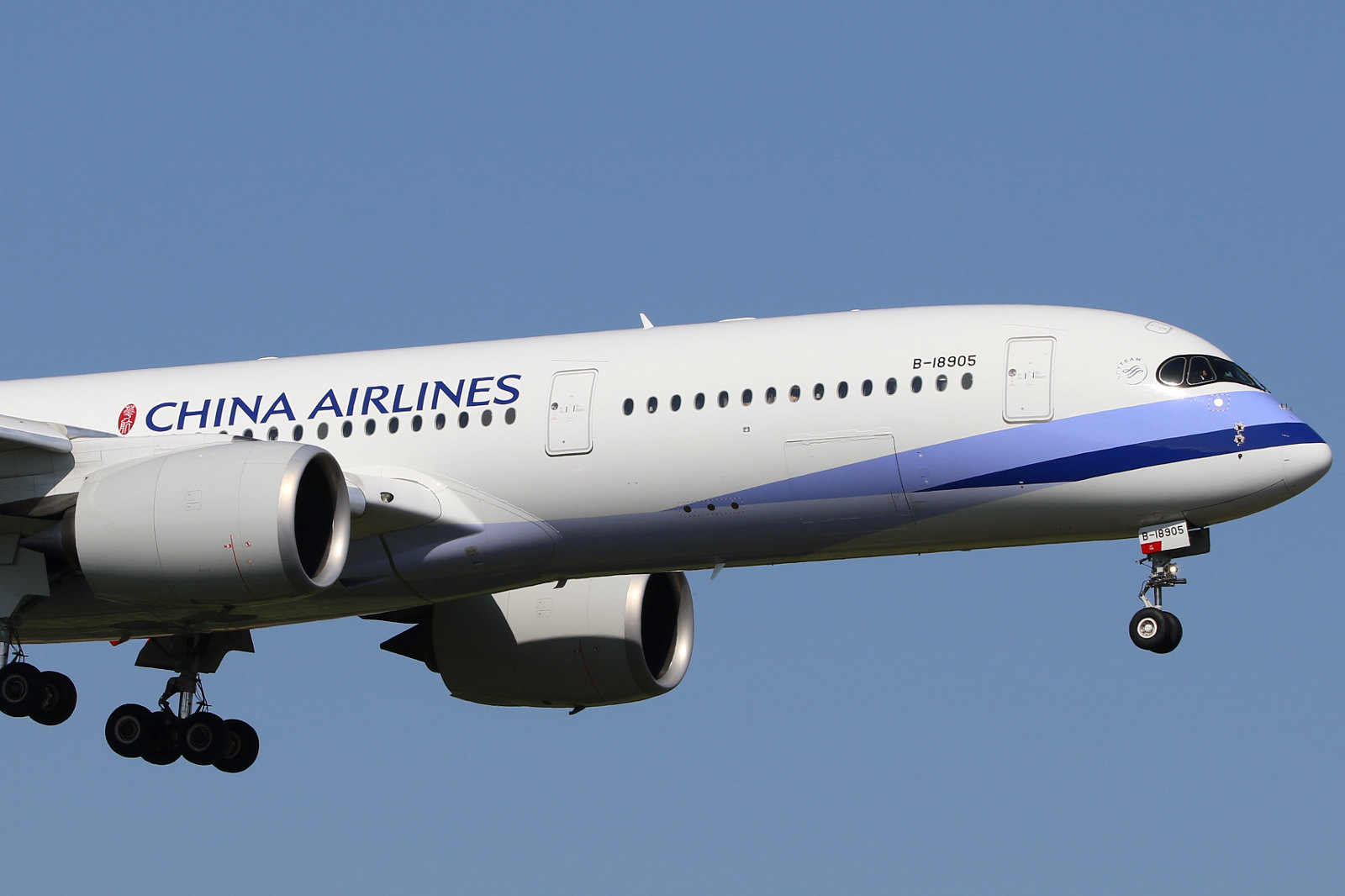A passenger aircraft, prominently situated in the center of the image, is depicted against a vivid, cloudless blue sky. The aircraft fills the frame from left to right, emphasizing its presence. Its landing gear is deployed, indicating it is in the process of landing, possibly at an airport. The plane is labeled with "China Airlines" along its side, accompanied by a logo. The fuselage features a design with various shades of blue including light blue, dark blue, and white, along with accents in red, gray, silver, and purple. The right side of the aircraft is visible, showcasing the cockpit window, passenger windows, doors, and part of the wing. The overall setting suggests it is taken outdoors in broad daylight.